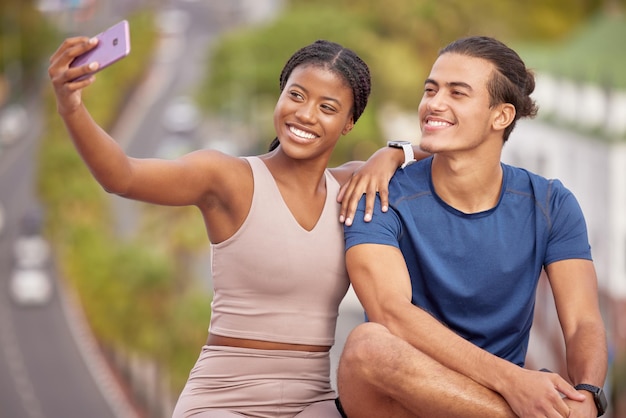In a bustling city park, two individuals sit closely on a bench, framed by a backdrop of blurred greenery and distant roads. Central to the image, the African-American woman, dressed in a pink tank top and matching yoga pants, extends her left hand affectionately to rest on the shoulder of the man beside her, while her right hand holds a purple smartphone to capture their smiling faces in a selfie. The man, sporting a blue short-sleeve t-shirt and his hair styled back into a sleek ponytail, relaxes with one leg crossed over his knee. Notably, the woman wears a white watch on her wrist, which is visible on the man’s shoulder, while the man dons a black smartwatch. Their joyful expressions and synchronized attire create a vibrant contrast with the tranquil, verdant park setting blurred in the background.